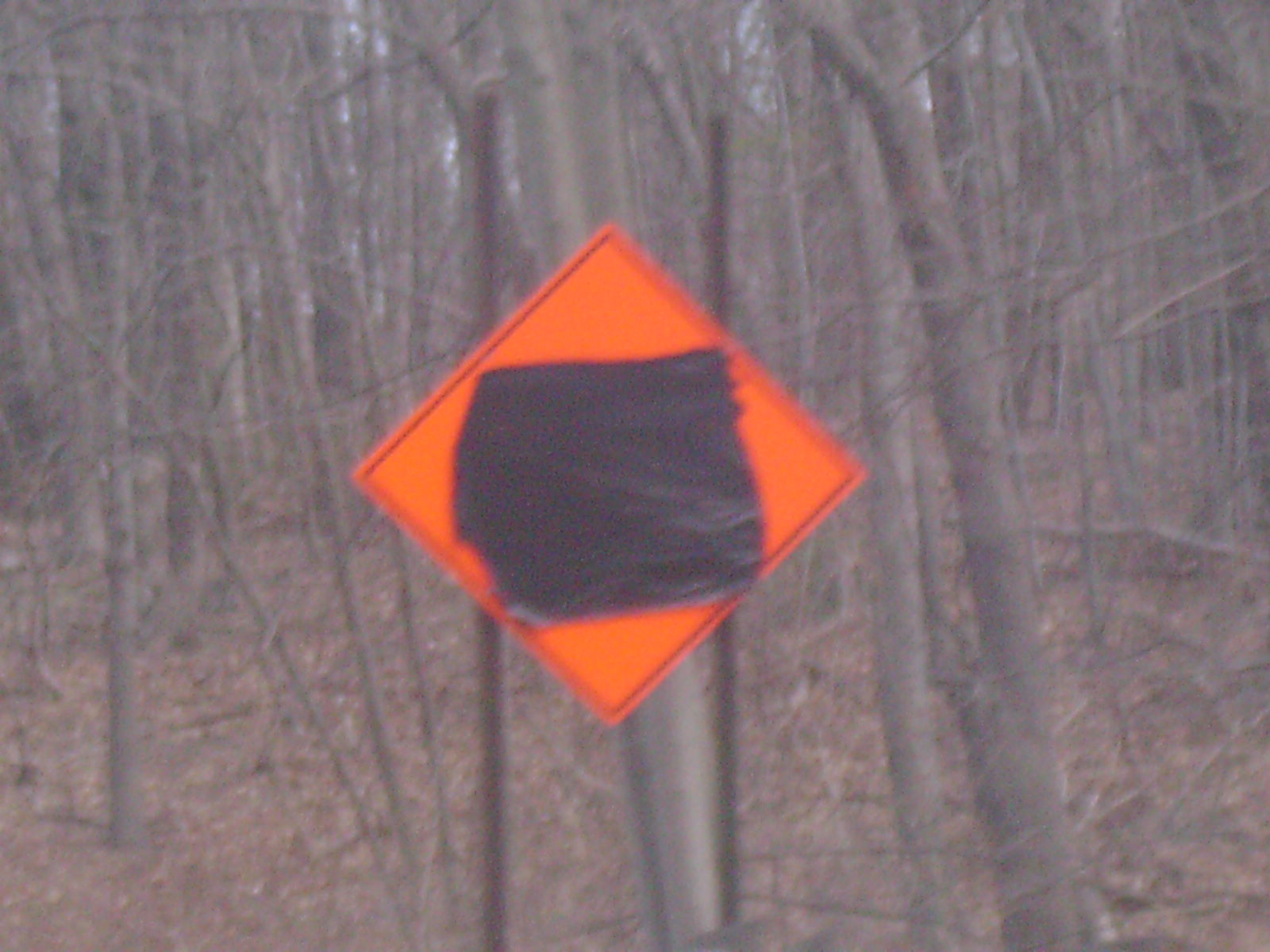A grainy photograph captures a diamond-shaped orange sign affixed to a tree. The sign, encased in a thin black border, is oddly obscured by a piece of black material that covers its central message or symbol, rendering it unreadable. Surrounding the sign is a barren, wooded area; leafless trees stand starkly against the overcast backdrop, contributing to the image's somber, desolate atmosphere.